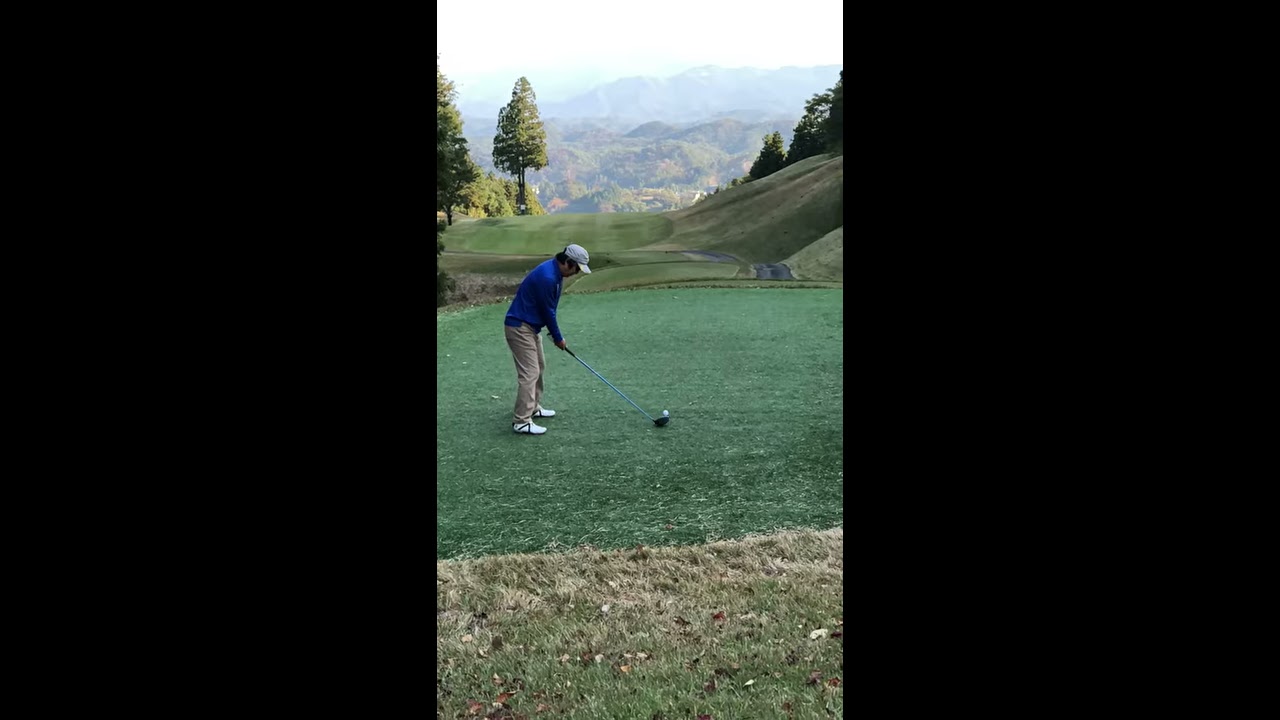A man is playing golf, positioned toward the right side of a vertically-oriented image. He wears a blue long-sleeve shirt, a white hat, and white shoes, with his feet shoulder-width apart and poised to hit a white golf ball with his long, silver, and dark-bottomed golf club. His beige khakis complement his outfit, and his black hair is visible beneath his hat. The golfer stands on a well-manicured green with patches of browner grass and scattered leaves in the foreground. To the right, a hillside ascends towards a roadway for golf carts, woven into the undulating landscape. In the background, lush green mountains and tall trees frame the scene, set against a backdrop of blue sky and white clouds. The detailed, vertical image is bordered by black on both sides, adding emphasis to the serene golfing moment.